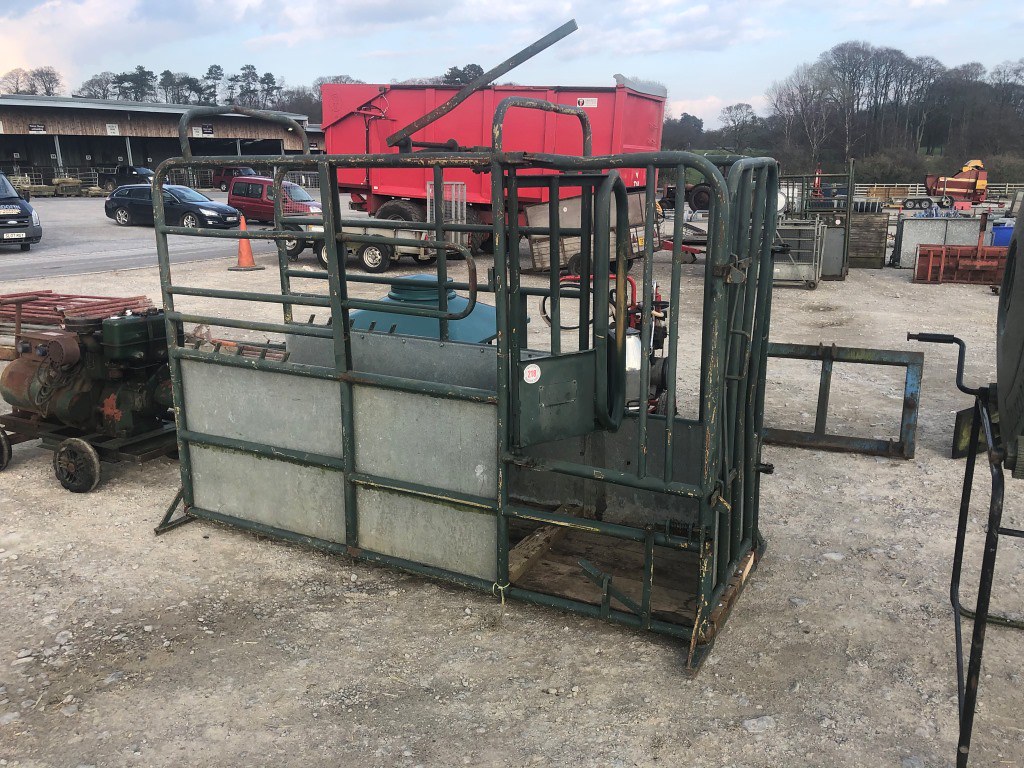The photograph reveals a cluttered industrial yard with various pieces of machinery, equipment, and debris, set against a backdrop of a large, possibly warehouse-like building, under a clear blue sky with scattered clouds. In the foreground, there is a distinctive narrow green metal chute, commonly used by cattlemen for branding stock, though it appears incomplete and weathered. Adjacent to it is a red bin-like structure from a pickup truck and a green generator mounted on a wheeled cart. Scaffolding, heavy machinery, and industrial containers are scattered around the area, displaying signs of rust and dirt. The ground is a packed, sandy surface with rocks, typical of an industrial setting. The background features parked cars, including black, maroon, and blue vehicles, and tall trees peeking over the buildings, which consist of warehouses or storage facilities. The entire scene gives off a sense of disuse and rugged utility, emblematic of a bustling yet cluttered industrial yard.